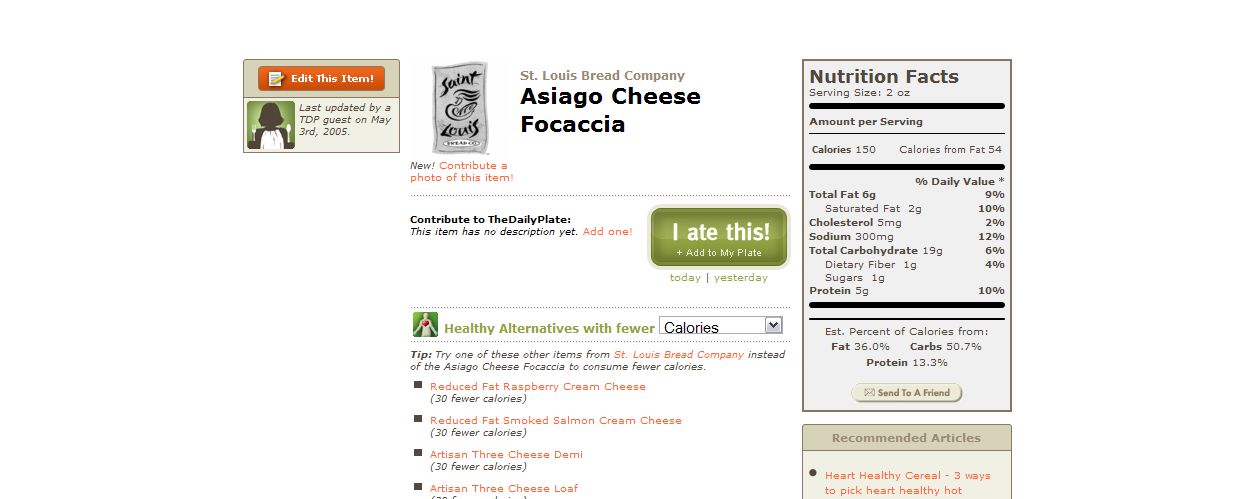The image showcases a detailed nutrition facts label for a food product. On the right-hand side, it prominently displays the heading "Nutrition Facts." Below this, it lists "Serving Size: 20 oz" followed by "Amount Per Serving." The caloric content is broken down as "Calories: 150" and "Calories from Fat: 54." Further down, there is the notation "Percent Daily Value*" with an asterisk, indicating the presence of footnotes or additional information.

On the left-hand side, the label provides a comprehensive breakdown of the nutritional components. It begins with "Total Fat: 6g" and "Saturated Fat: 2g," followed by "Cholesterol: 5mg" and "Sodium: 300mg." Next, it lists "Total Carbohydrate: 19g," which includes "Dietary Fiber: 1g" and "Sugars: 1g." Finally, the label concludes with "Protein: 5g."

The information is meticulously presented to inform consumers about the nutritional content of the serving, aiding in dietary choices.